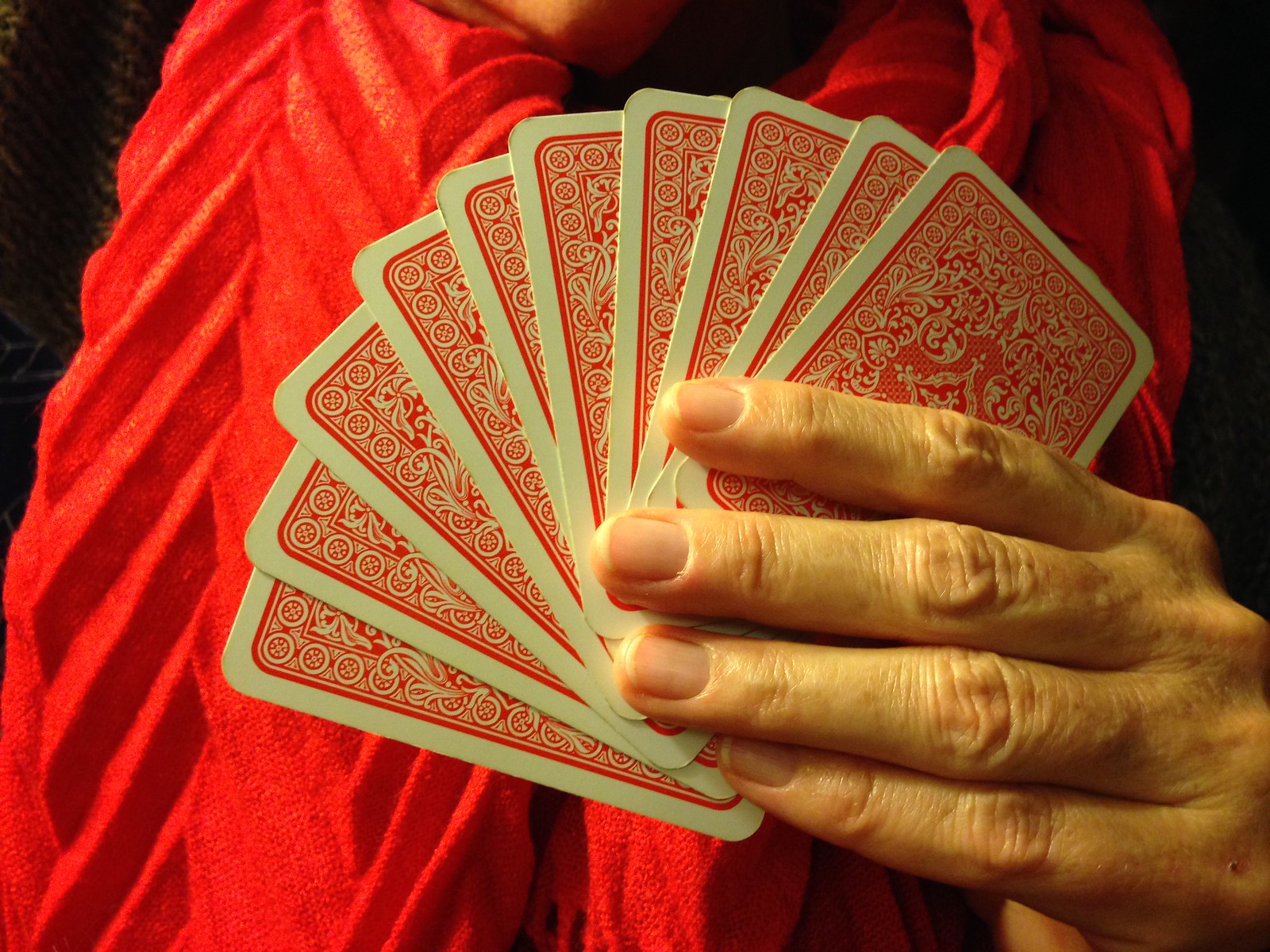Indoor color close-up photograph depicting an older person's left hand holding a fanned-out hand of 10 cards. The person appears to be in their late 30s or early 40s, with a light skin tone. The back of the cards, not the numbered side, are visible, displaying a detailed floral red print. The person's four fingers are clearly shown coming in from the left edge, though the fingertips are slightly blurry. The individual's fingernails are neatly trimmed, and they are not wearing any rings.

In the background, the person is seen wearing a distinctive ruffled red jacket or sweater, characterized by slightly diagonal folds on the sleeves and chest. A hint of the person's neck is visible along the top edge of the image. The upper left, lower, and upper right portions of the background are entirely black, providing a stark contrast to the vibrant red elements in the photograph. The overall focus of the image is sharp on the back design of the cards, emphasizing their intricate pattern. The photograph is devoid of any text or print, solely capturing the moment of a person presenting their hand of cards.